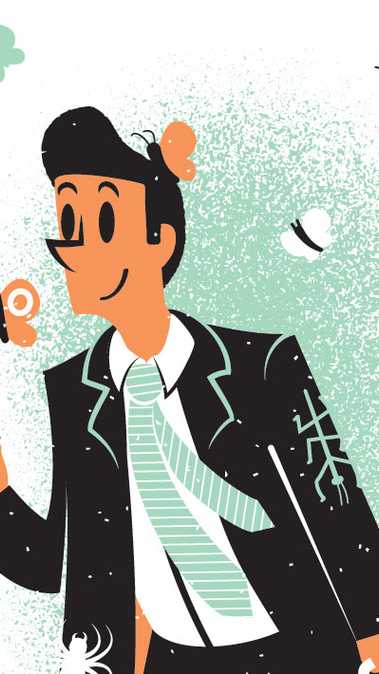The image is a detailed, digitally rendered drawing of a cartoon-like man oriented to the left. The man, who has dark black hair with a straight hairline and a tall front tapering towards the back, sports a black suit adorned with light teal stripes along the collar and shoulders, complemented by a white shirt and a light teal tie with white stripes. Mounted on the back of his head is an orange butterfly with a black body and black antennas. The man appears to be smiling and facing slightly left but looking forward. Several butterflies of varying colors—orange, white, and blue—are flying around him, including one white butterfly with a black body and another orange butterfly with distinctive markings. In the background, a green paint blotch splatters across a white wall. Notably, a light green bug with multiple legs and a long tail is depicted walking down his right arm, while the silhouette of a white scorpion-like creature is visible climbing up the bottom left of his suit.